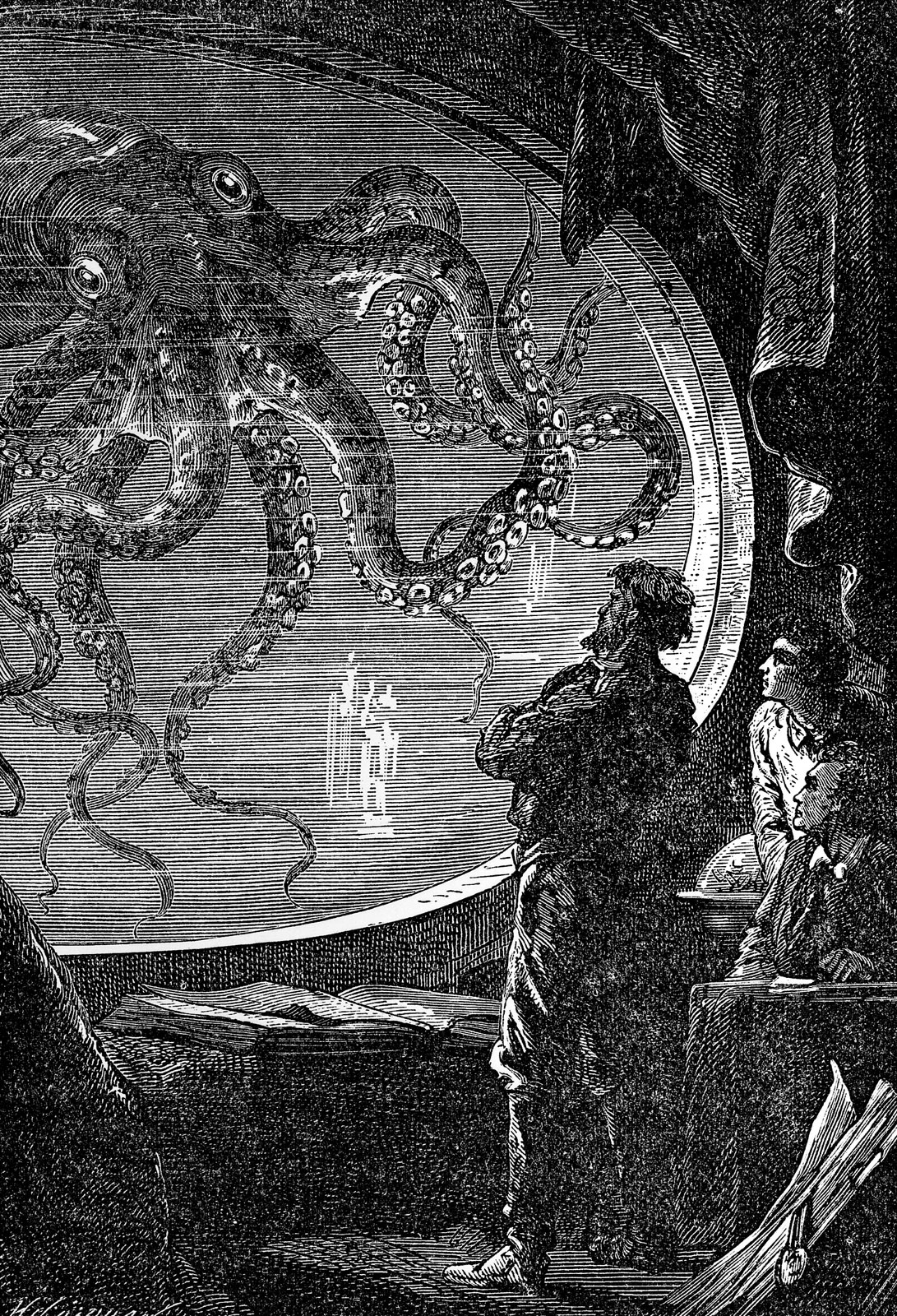The image is a detailed black and white sketch encapsulating a dramatically eerie scene. In a vertically rectangular frame, three men are situated in a dark room and intently observing a colossal octopus through a large, horizontal oval window. One man stands proudly near an open, oversized book, while the other two men sit beside him, all focused on the creature outside. This room is furnished with scholarly objects including a globe and a massive drapery hanging above the window. The octopus, with its enormous eyes, gazes back at the men, creating an atmosphere filled with curiosity and foreboding. The intricate illustration resonates with a vintage, hand-drawn quality, reminiscent of early daguerreotype styles, adding to the mystique of the scene.